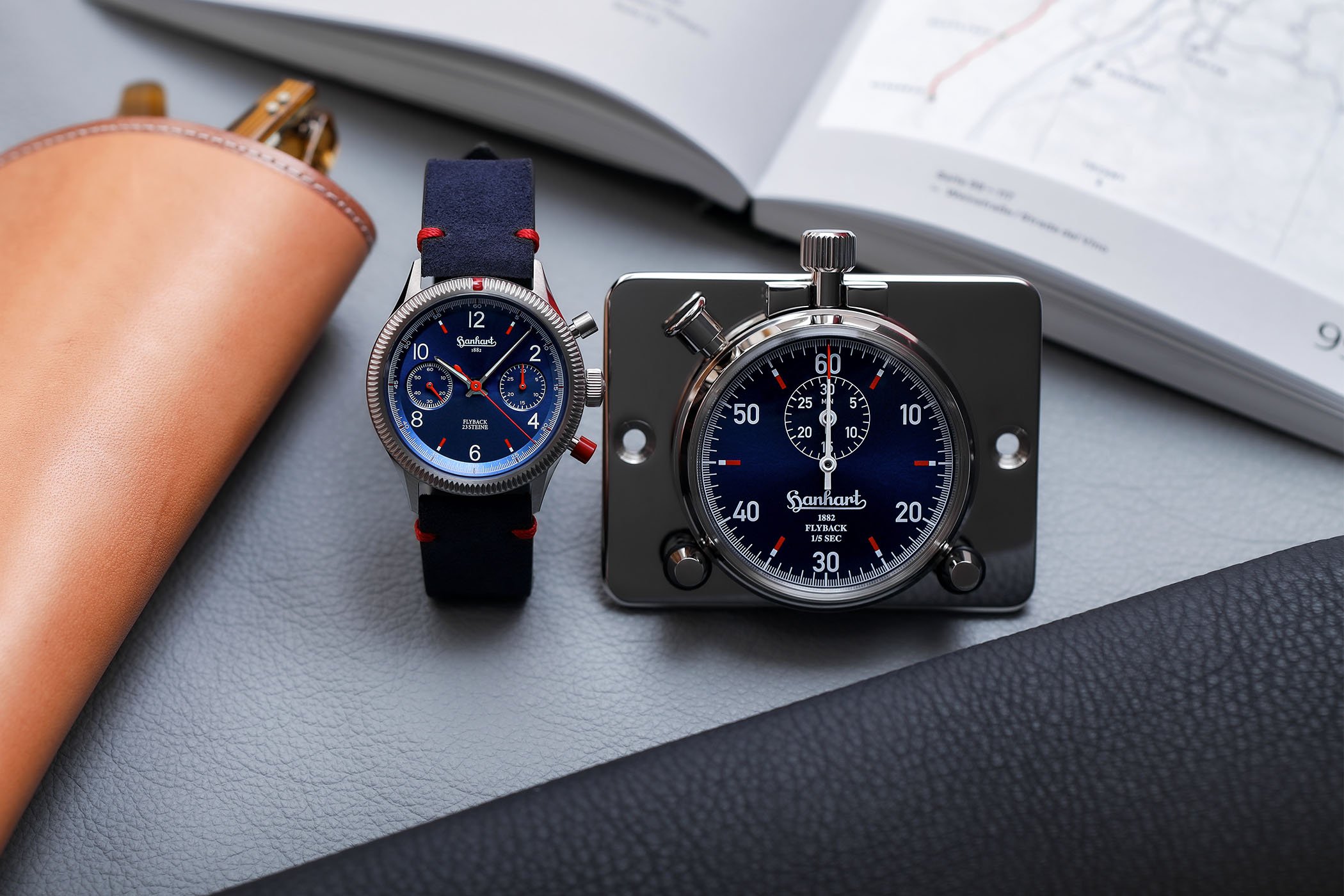In the image, a meticulously arranged ensemble of luxurious items is displayed on a sleek gray table. Dominating the arrangement is a sophisticated watch featuring a dark blue strap and a striking face with silver accents, red and white elements, and numerals for 12, 2, 4, 6, 8, and 10. Adjacent to the watch is a dark gray timer with a black face, prominently displaying the numerals 10, 20, 30, 40, 50, and 60, crafted by Bernhardt. A rich brown leather case, partially open to reveal a matching pair of glasses, sits to the left of the watch. Overhead, a book with detailed diagrams suggests someone is engaged in study or planning. This appears to be a professional product photo, possibly showcasing a coordinated collection, emphasized by the refined lighting and composition. The items rest atop a leather desk mat, adding a touch of elegance to the overall scene.